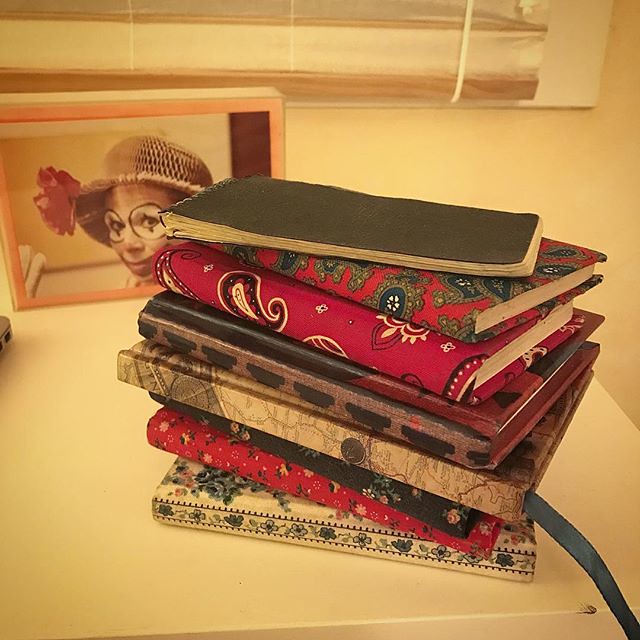In the image, there is a stacked array of books on a sleek, contemporary white night table. The books display varying covers, some adorned with unique fabric materials such as paisley and red bandana prints, giving them a handcrafted and decorative appearance. The topmost book is a spiral notebook with a black cover. Among the books, a few have hardcovers, one of which has a ribbon bookmark poking out on the right. 

Behind the stack, a photograph stands out in an orange, shadow box-like frame. The photo captures a figure dressed as a clown, characterized by striking makeup featuring white eyes with vertical black accents and red lipstick. The clown wears a paper hat adorned with a red flower. The background also reveals a wooden window treatment and the bottom of a white-painted window frame. The scene feels intimate and cozy, with the books and the distinct clown picture accentuating the unique atmosphere.